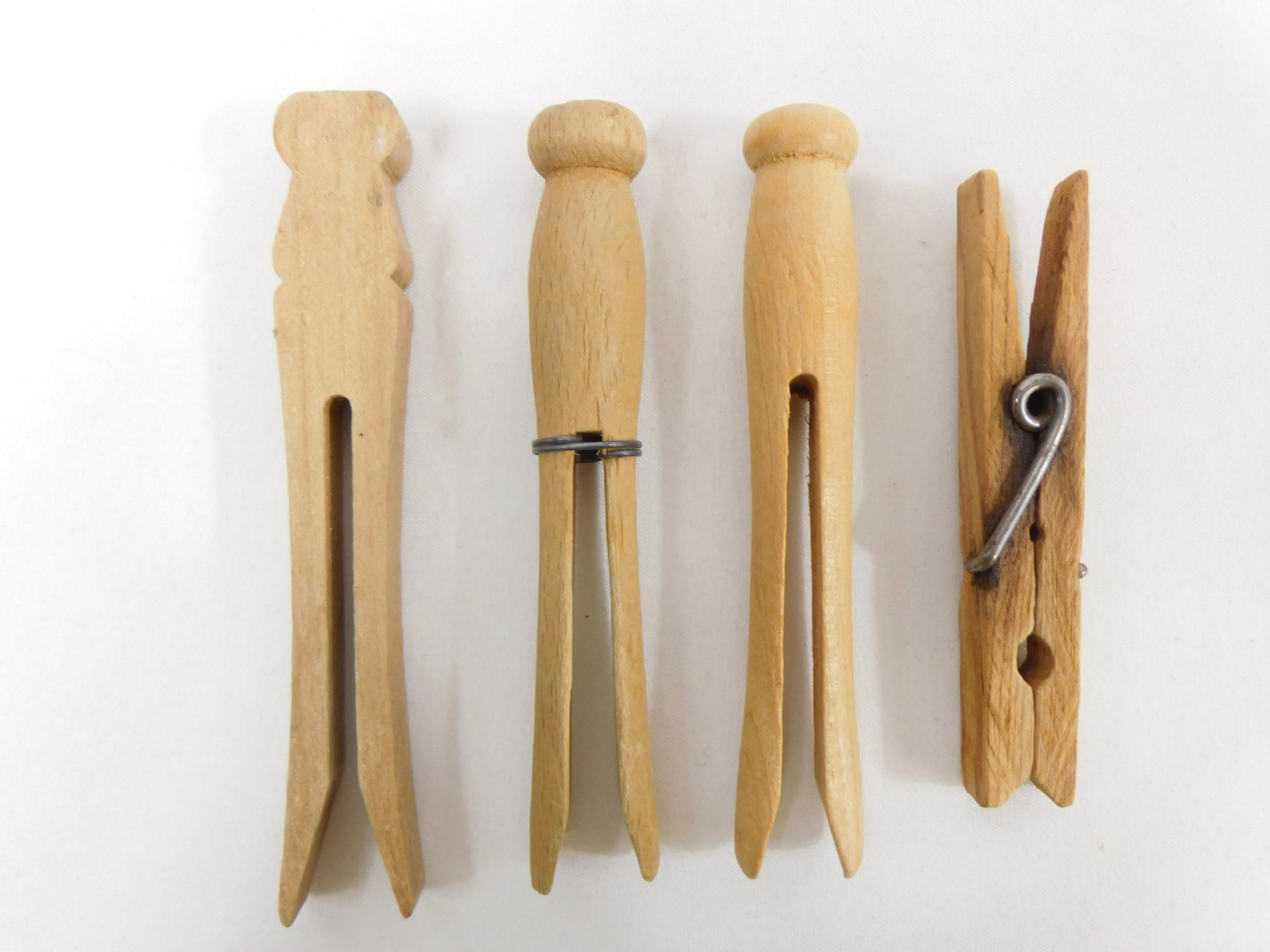The image showcases a progression of four distinct clothespins, each varying slightly in design, all set against a white surface with their shadows cast beneath them. The first clothespin on the far left is a longer, one-piece wooden pin with a V-shaped notch at the bottom and decorative indents on the sides, resembling a duckbill. Next to it, the second clothespin features a similar single-piece design with a gently sloping V-shaped opening, accentuated by a gray metal spring coiled around its middle, giving it a more open appearance. The third clothespin resembles the second one but is slightly shorter, with its notch starting higher and lacking the metal spring. The final clothespin on the far right is a modern design with a spring mechanism that joins two separate legs, forming a triangular top that opens when squeezed. This sequence beautifully illustrates the evolution from traditional single-piece wooden clothespins to the contemporary spring-loaded versions.